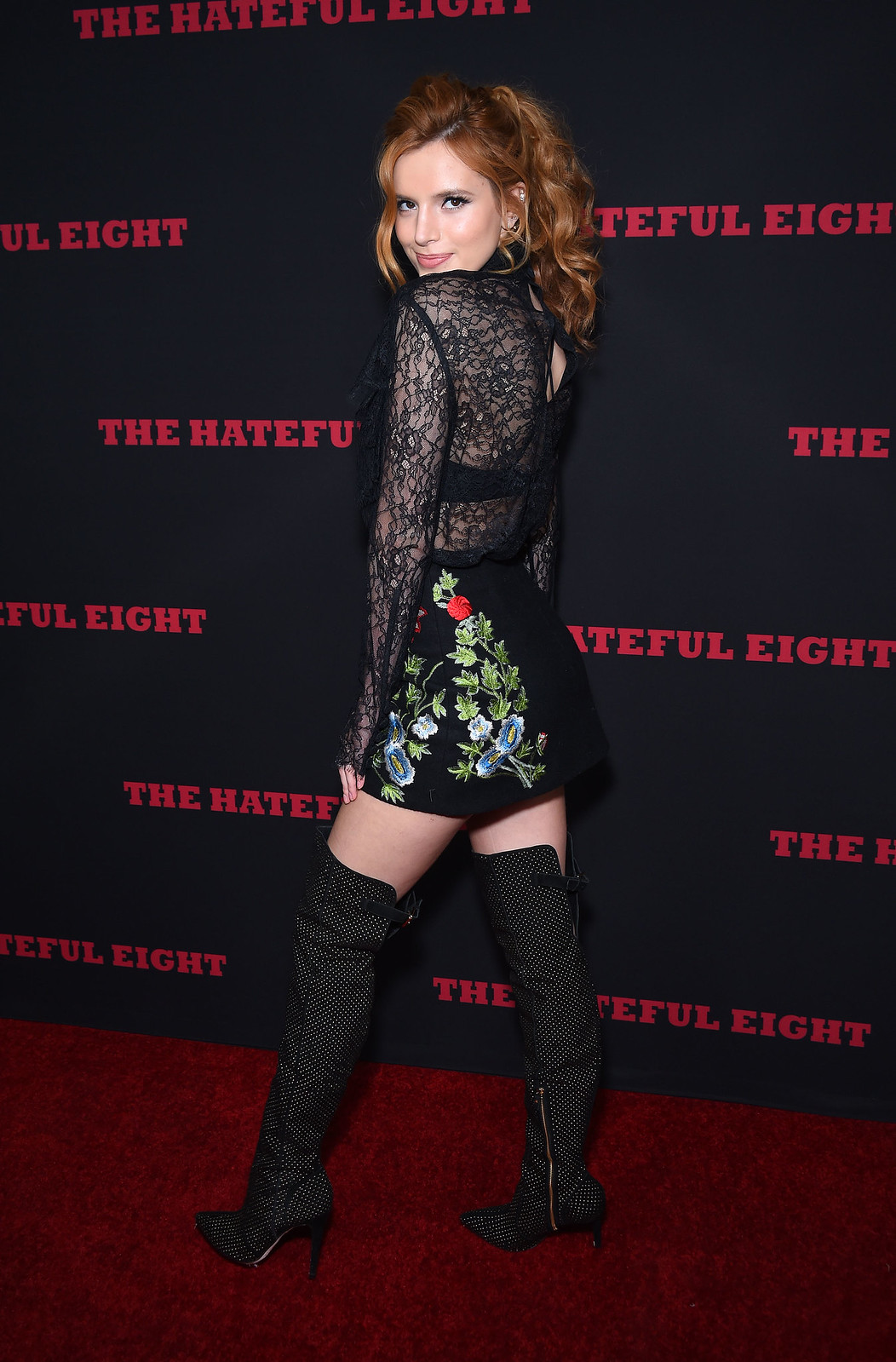This is a detailed photograph of actress Bella Thorne posing on the red carpet at the movie premiere of "The Hateful Eight." Bella is turned towards the back, gazing over her shoulder with a smile that highlights her pronounced cheekbones. Her reddish-brown, wavy hair cascades down her back. She is dressed in a lacy black top that's see-through, revealing a black bra underneath, and paired with a short black skirt adorned with embroidered patterns of red and blue flowers and green leaves. Completing her look are high-heeled black boots speckled with white, extending just past her knees. She stands confidently on the red carpet with the backdrop showing "The Hateful Eight" repeatedly written in bold red letters. The event commemorates Quentin Tarantino’s cowboy movie, which starred Kurt Russell among other notable actors.